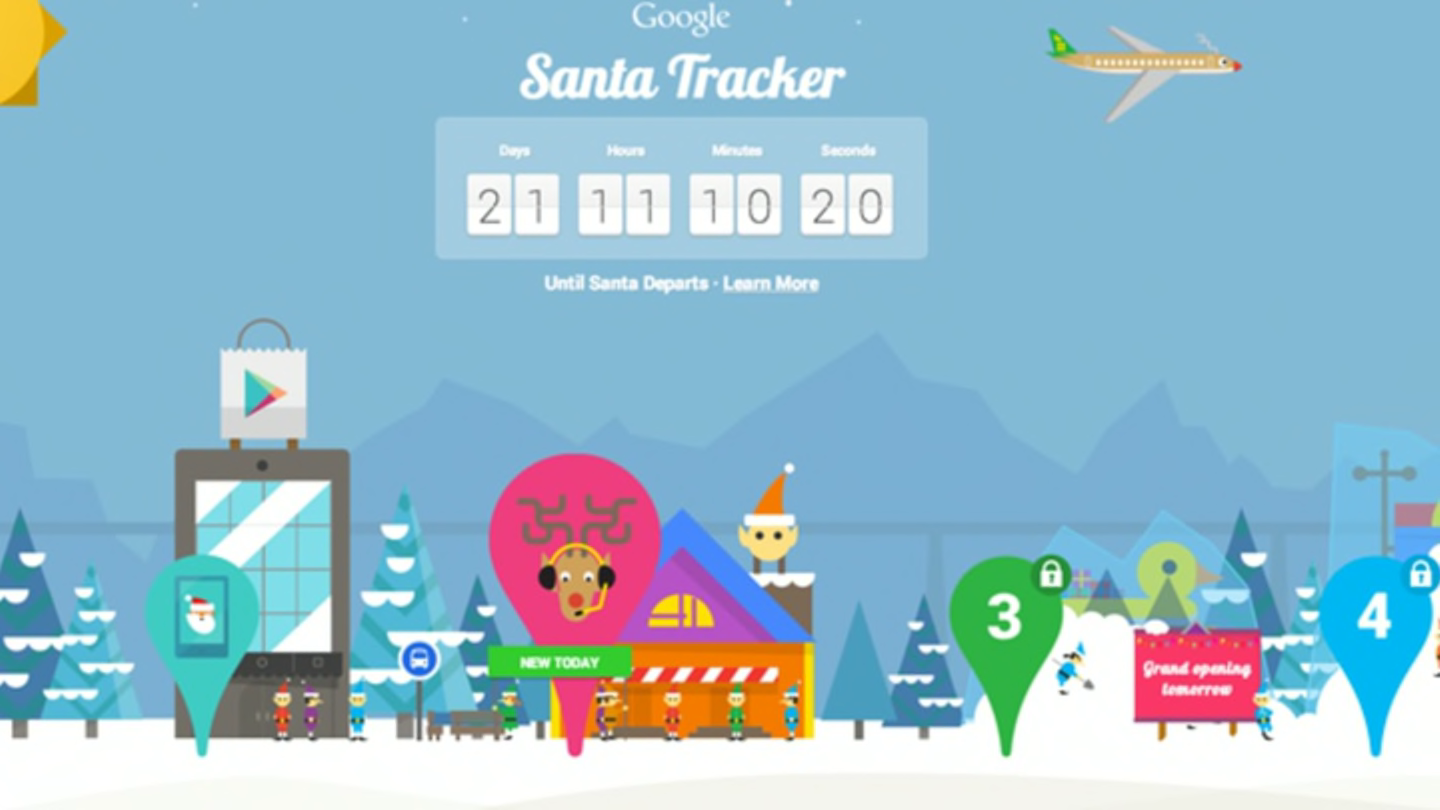The image is a detailed screen capture from Google’s Santa Tracker. It features a whimsical, festive scene set against a light blue and white backdrop, with snow-capped mountains in the distance. To the left side, a golden sun shines brightly. Dominating the sky is a golden, green, and silver airplane adorned with a reindeer head, complete with a red nose.

In the foreground, a vibrant North Pole setting unfolds. Blue snow-covered trees stand prominently before a large gray object resembling a smartphone, decorated with blue and gray squares. Beside it is a white Google shopping bag icon with a teal and pink play button and a silver handle. Nearby, a teal icon with a cell phone graphic shows a red and white Santa head.

Three elves – one in red, one in purple, and one in blue – stand near the huge gray phone, beside a blue and gray bus stop sign. A green-clad elf is visible next to a pink location pin adorned with a reindeer head, headset, and a green box that reads "New Today."

A colorful house displaying hues of purple, blue, yellow, and orange is surrounded by elves color-coordinated to match their environment: purple, orange, green, and blue outfits. Their skin tones are peach.

Another location pin, this one green, bears a white number three and a padlock symbol. An elf in blue shovels snow nearby. Close to a red sign adorned with Christmas lights which announces "Grand Opening," an elf in blue leans against it, with another blue location pin marked with a white number four and a padlock symbol visible nearby.

At the top of the image, above the mountain range, a banner reads, "Google Santa Tracker: 21 days, 11 hours, 10 minutes, 20 seconds until Santa departs. Learn more."

The scene encapsulates the playful and interactive spirit of Google’s Santa Tracker, with each detail contributing to a lively and engaging holiday tableau.